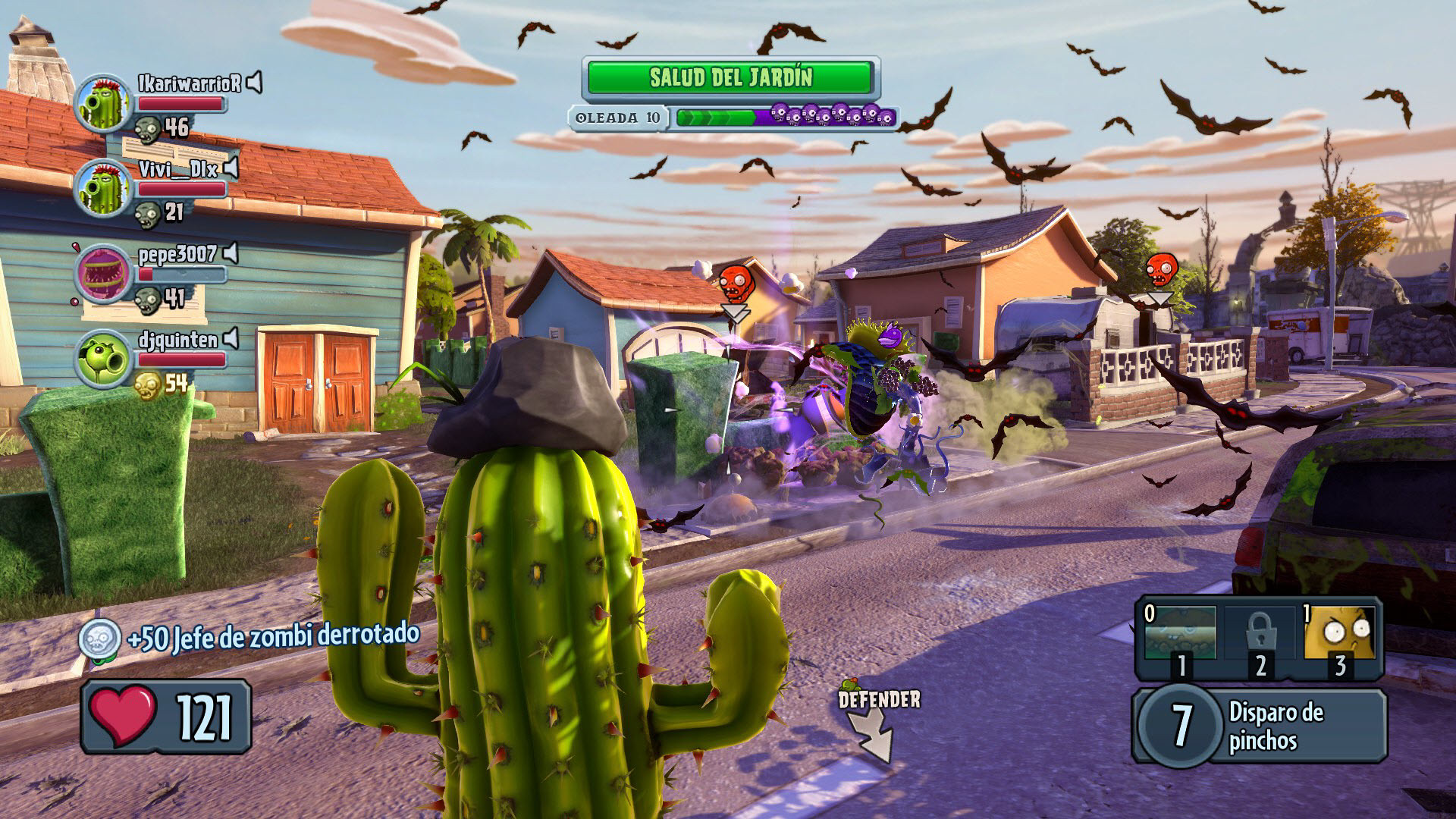This image appears to be a screenshot from the video game "Plants vs. Zombies," featuring a vibrant and exaggerated cartoonish art style. The scene is set on a street amidst apparent chaos and destruction, possibly from a recent explosion, indicated by debris and a damaged vehicle. Prominently featured in the foreground is a cigar-smoking cactus, adorned with a hat, walking down the street. In the lower left-hand corner, a heart icon displays "100/121," alongside text in Spanish. Above the heart, there's a circular icon of a skeleton with the text "+50 jefe de zombie Dorota Dora Dara Toto."

Several zombies populate the street, heightening the sense of mayhem. Additionally, numerous bats with red eyes fill the sky, adding to the eerie atmosphere. At the top of the image, the text "Salud del Jardin" is visible, framed by cartoonish clouds, completing the whimsical yet chaotic street scene overrun by zombies.